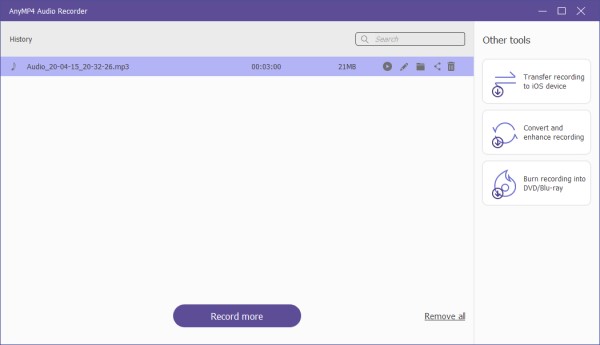The image depicts a user interface with a variety of elements organized as follows:

At the top, there is a purple rectangular banner, which contains text on the left side reading "Any MP4 Audio Recorder" in white font. To the right of this text is a white-bordered square with an 'X' inside it, framed by a gray background.

Below this banner, on the right side, there is a gray section labeled "History" in bold black font with a capital 'H'. Adjacent to this label is a search box, outlined in a darker gray with a lighter gray interior. Inside the search box, there is a gray magnifying glass icon next to the word "Search," also in gray with a capital 'S'.

To the left of the gray section, the background lightens slightly, bearing the label "Other tools" in bold black font. Under this heading are three white-background rectangles with black text. The first rectangle reads "Transfer recording to iOS device," the second says "Convert enhanced recording," and the third indicates "Burn recording into DVD/Blu-ray."

At the very bottom of this interface, there is an underlined black text link that says "Remove all." Just above this link, there is a prominent purple oval button with the text "Record more" in bold white font with a capital 'R'.

Above these elements, within a light purple border, there is a file name displayed in black text: "Audio_20-04-15_20-32-26.MP3." Alongside the file name, smaller text displays the file duration "00:03:00" and the size "21 MB."